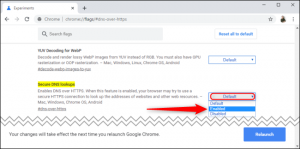This image is a screenshot of a website with a white theme. The website is displayed on a browser with only one tab open. Despite zooming in, the text within the small elements remains hard to read. The interface shows a continuation of the white background through the entire screen. Notably, at the top left corner, there is a blue icon beside the website’s name. 

Navigating through the page, you will encounter several paragraphs and boxed text. On the left side of the screen, towards the bottom, a section is highlighted in yellow. Further down, in the lower-middle area, a significant portion of text is emphasized with a wide red arrow, suggesting its use in a teaching or instructional context. Additionally, a word near the top of the page is circled in red, drawing attention to it. Finally, there is a blue button visible at the bottom of the page.